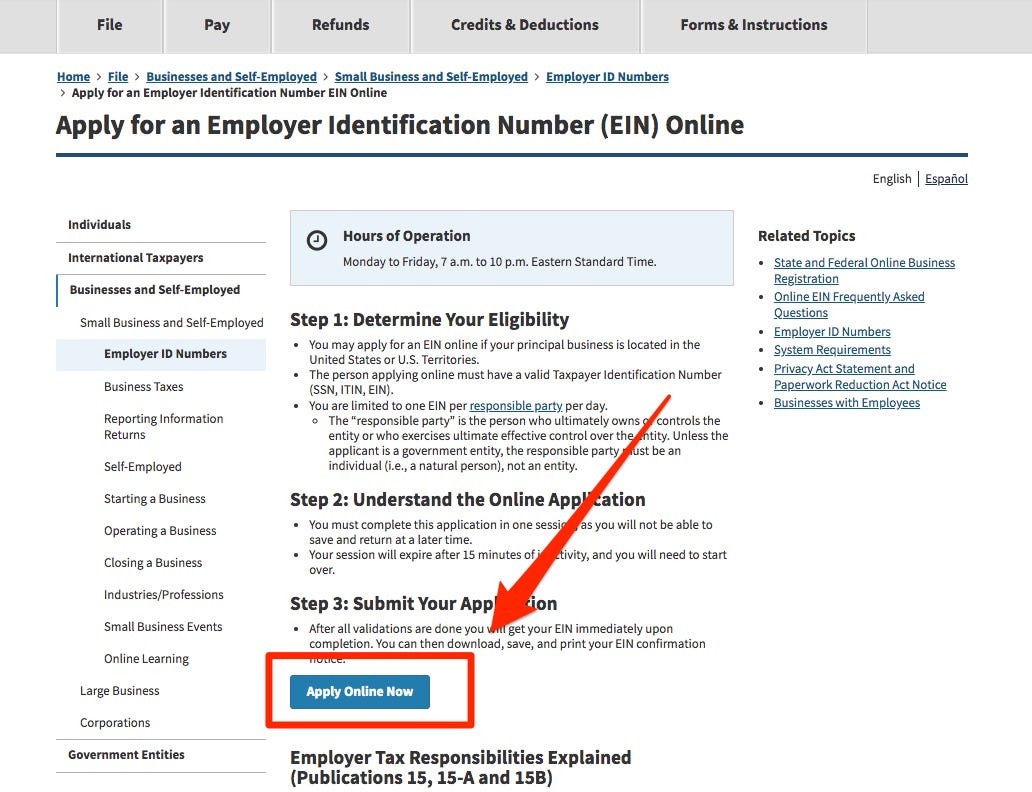The government webpage for applying for an Employer Identification Number (EIN) features various sections and options. At the top, bold headers indicate categories like "Home," "File," "Business," and "Self-Employed." Below, a notification highlights the option to apply for an Employer Identification Number online. A blue information box indicates the hours of operation: Monday to Friday from 7 a.m. to 10 p.m. Eastern Time.

On the left side of the page, a menu offers links for various categories such as:

- Individuals
- International Taxpayers
- Business/Self-Employed
- Small Business/Self-Employed
- Employer ID Numbers
- Business Taxes
- Reporting Information Returns
- Starting, Operating, and Closing a Business
- Industry Professions
- Small Business Events and Online Learning
- Large Businesses/Corporations
- Government Entities

In the center of the page, important instructions guide users through the application process. The first step is "Determine your eligibility," with explanatory text beneath it. This is followed by "Understand the application," labeled as step two. The steps are marked with giant red arrows pointing towards a prominent blue button labeled "Apply Online Now," surrounded by a large red box. Step three is "Submit your application."

Toward the bottom of the page, it details "Employer Tax Responsibilities Explained" with references to publications 15, 15-A, and 15-B. 

In the top right corner, the site offers language options, "English" or "Español," followed by a "Related Topics" tab containing additional resources.